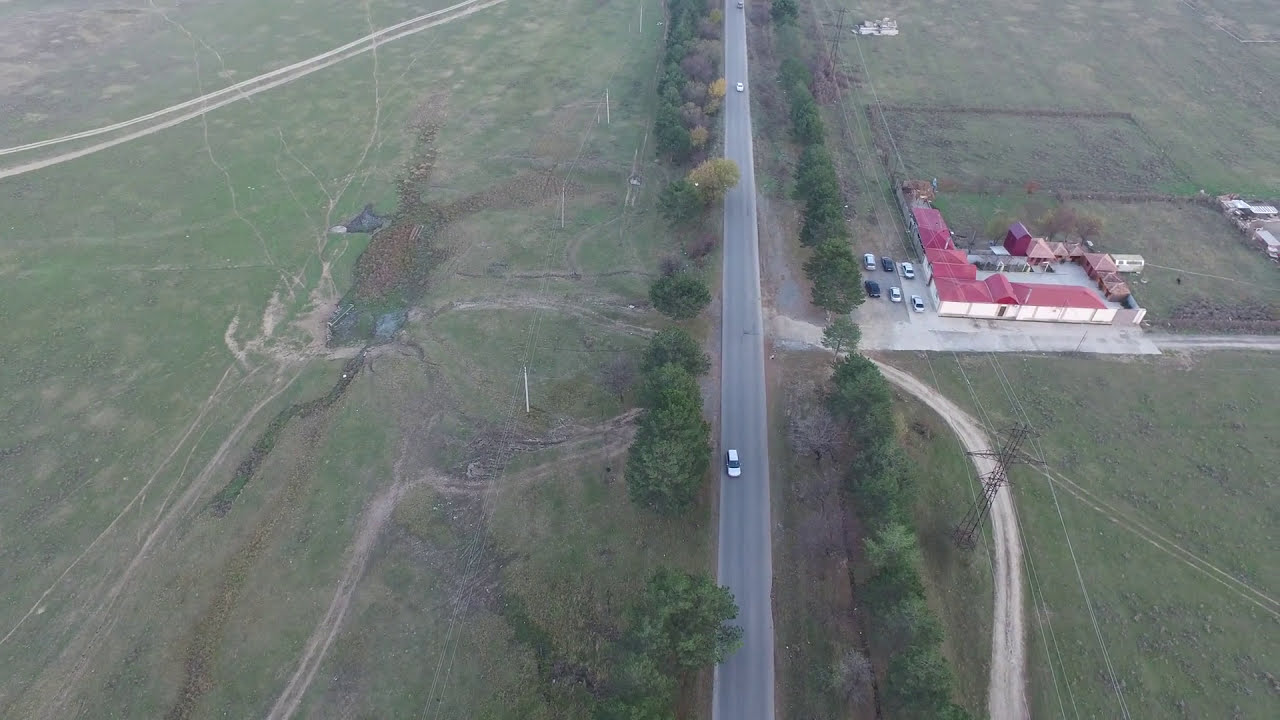The aerial image captures a two-lane asphalt highway flanked by lush trees, some dotted with yellow leaves, and a few barren ones. Two white cars travel on the highway, one in each direction. Power lines run along both sides of the road - on the right, they are supported by dark metal poles, and on the left, by white poles. Adjacent to the highway on the right side, there is a white-walled building with a red roof, likely a diner or a farmhouse, framed by a concrete parking lot with six cars. Four of these cars are white, two positioned at the front and two at the back, while two dark-colored cars are also visible. On the left side of the image, the landscape transitions into a grassy field with erratic trails and a small, foggy, and waterlogged patch.